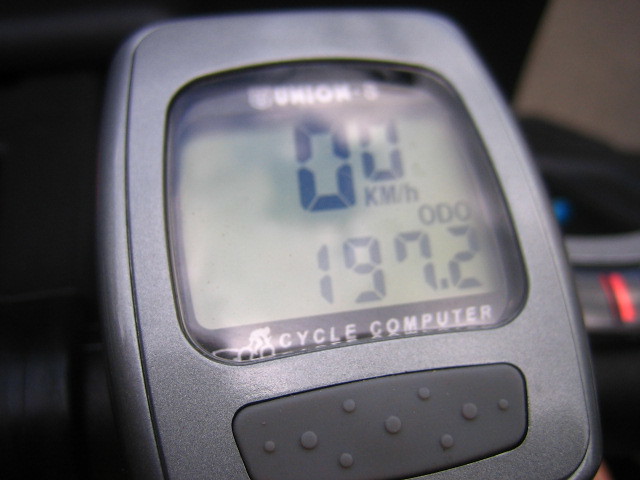This is a color photograph featuring a sleek, gray digital device. The surface of the device is seamlessly smooth, exuding a modern and minimalist design. Centrally positioned is a square digital display with rounded corners, bearing a slight glare that partially obscures the screen. Nevertheless, the display prominently reads "Union" at the top in crisp white text, and "Cycle Computer" at the bottom.

The digital screen's main element is a large numerical zero, accompanied by a smaller zero with "KM/h" beneath it, indicating the speed measurement in kilometers per hour. Below this, a numerical value of 197.2 is displayed, possibly representing distance or another metric.

Positioned under the digital screen is a dark gray rectangular bar, adorned with several raised gray discs, suggesting control buttons for device navigation. The background is indistinct and blurred, predominantly gray on the right side, featuring horizontal gray strips and a strikingly bright red vertical strip that adds a pop of color to the otherwise monochromatic scene.